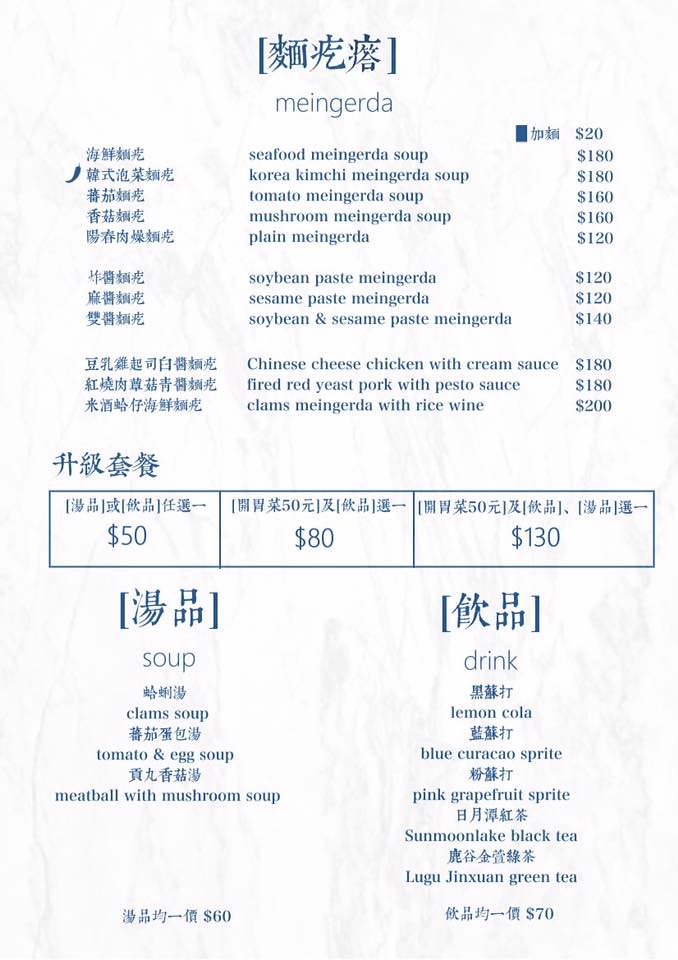This is a detailed description of a menu page from an Asian restaurant featuring both Asian pictographic symbols and English text with accompanying prices denoted in dollars. At the top, the word "MEINGERDA" is prominently displayed. The menu primarily lists various "Maguirda" dishes with their respective prices:

- Seafood Maguirda Soup: $180
- Korea Kimchi Maguirda Soup: $180
- Tomato Maguirda Soup: $160
- Mushroom Maguirda Soup: $160
- Plain Maguirda: $120
- Soybean Paste Maguirda: $120
- Sesame Paste Maguirda: $120
- Soybean and Sesame Paste Maguirda: $140

Additional main dishes include:
- Chinese Cheese Chicken with Cream Sauce: $180
- Fried Red Yeast Pork with Pesto Sauce: $180
- Clams Maguirda with Rice Wine: $200

Below these listings, there is a section containing more Asian symbols with prices displayed in boxes labeled $50, $80, and $130, possibly representing additional side dishes or small plates.

At the bottom of the menu, there's a selection of soups, with alternating Asian symbols and English text:
- Clam Soup: $60
- Tomato and Egg Soup: $60
- Meatball and Mushroom Soup: $60

The other side of the menu lists drinks, priced at $70 each:
- Lemon Cola
- Blue Carasauce Sprite
- Pink Grapefruit Sprite
- Sumon Lake Black Tea
- Wong's Yixian Green Tea